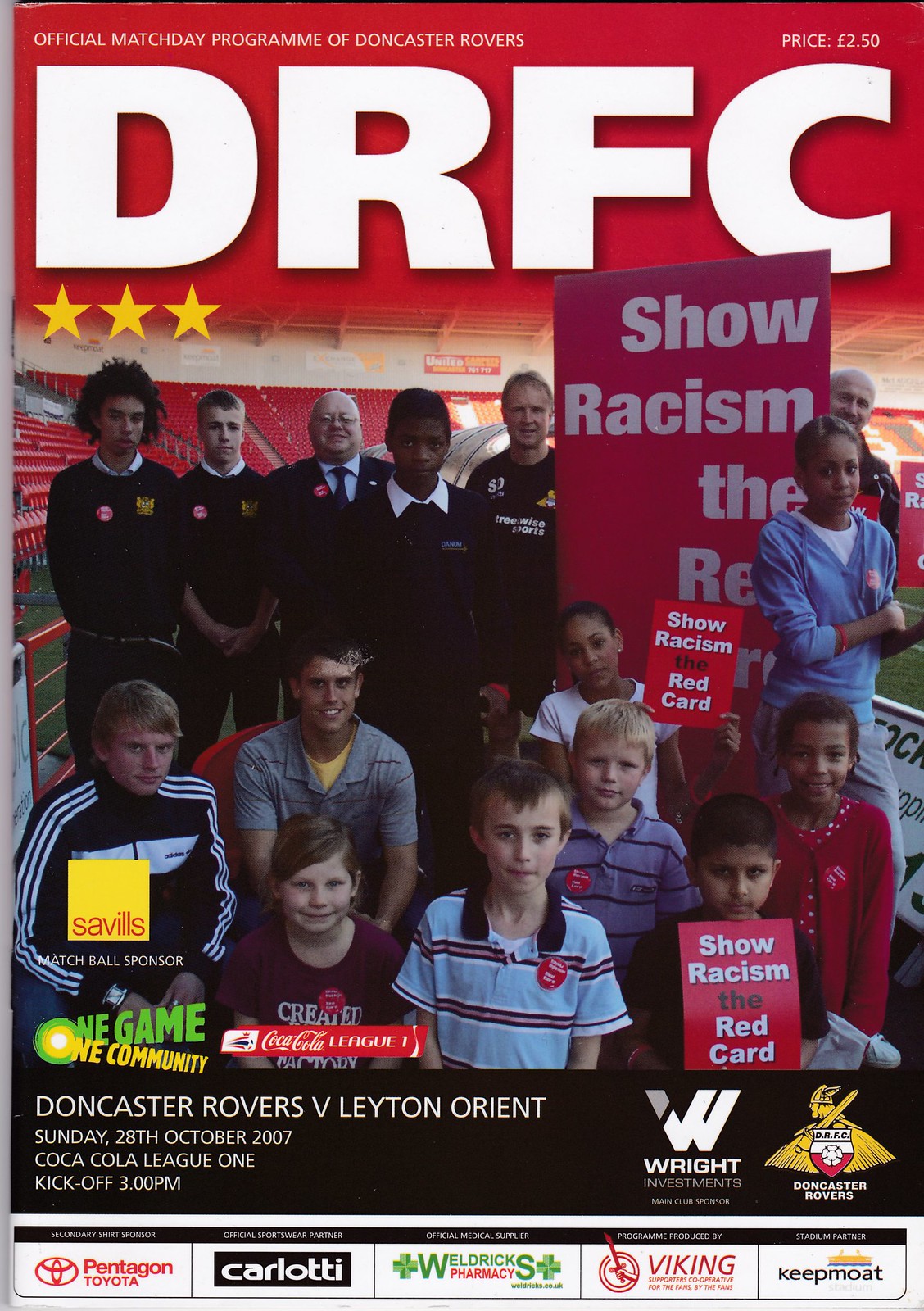The photo is the cover of the Official Match Day Program for the Doncaster Rovers Football Club (D.R.F.C.). The predominantly red-themed cover features a diverse group of individuals, including children and adults. The children are dressed in a mix of uniforms and casual clothing, all adorned with pins reading "Show Racism the Red Card." They are holding signs that echo the same anti-racist message. Positioned centrally in the image, the group is framed by a large, partially obscured banner in the background that also reads, "Show Racism the Red Card."

The top of the cover prominently displays the title "Official Match Day Program of Doncaster Rovers," along with a price of £2.50 and the club's acronym, D.R.F.C. Below the group, essential details about the soccer game are highlighted: "Doncaster Rovers vs. Leyton Orient, Sunday, October 28, 2007, Coca-Cola League One, kickoff at 3 p.m.” Further down, an array of logos for various sponsors are listed, including Seville's, One Game, One Community, Coca-Cola, Doncaster Rovers, Wright Investments, Pentagon Toyota, Carlotti, Weldrick Pharmacy, Viking, and KipoMote. The presentation and layout suggest that this cover aims to promote both the upcoming match and the crucial anti-racism campaign.